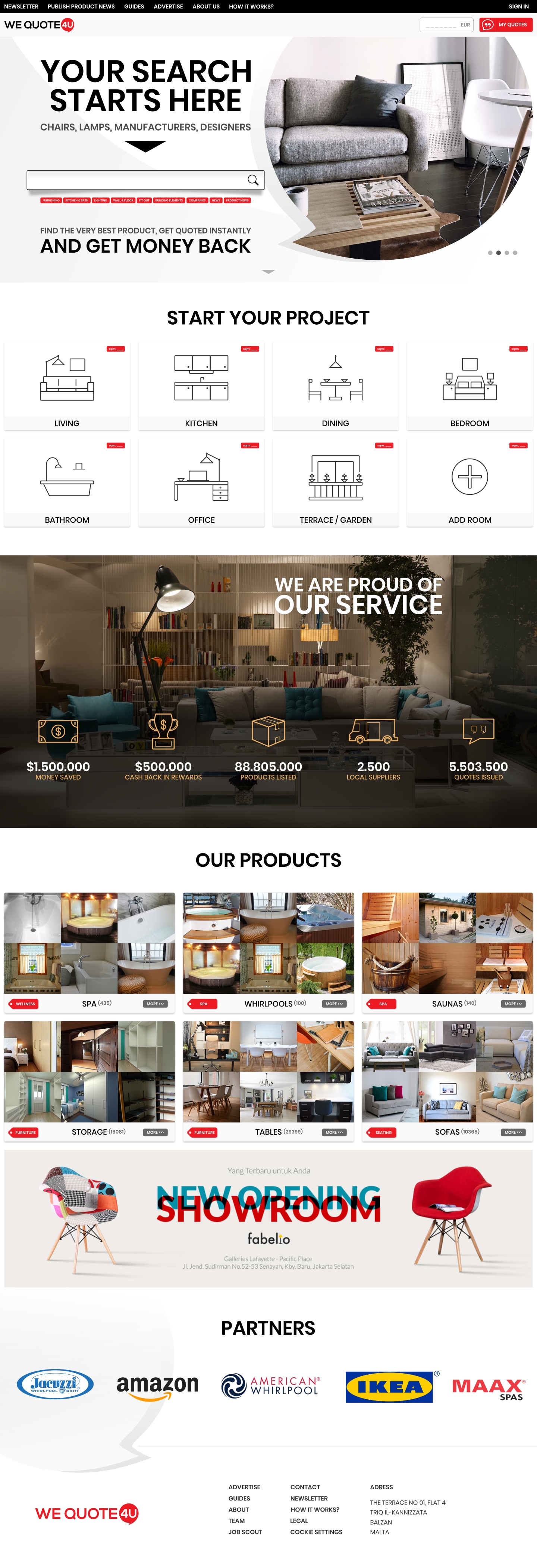**Website Screenshot of WeQuote4U**

**Header:**
The website’s header is in black and features multiple navigational links from left to right: Newsletter, Publish Product News, Guides, Advertise, About Us, How It Works, and Sign In. To the right of “Sign In” is a red box labeled "MyQuotes" in white font. Adjacent to "MyQuotes" is an outlined rectangular box with the text "EUR" indicating the European section of the site.

**Main Body:**
- **Introduction:** Bold text reading "Your Search Starts Here" is followed by smaller text listing categories: Chairs, Lamps, Manufacturers, Designers. An arrow directs users to a central search box.
- **Imagery:** The visual includes a couch, a table with a chair, a painting, a table with a mug and a magazine, and a rug underneath the table.
- **Call to Action:** Below the imagery, bold text reads "Start Your Project". To the left, phrases including "Find the Very Best Product," "Get Quoted Instantly," and "Get Money Back" emphasize the service’s benefits.

**Project Categories:**
- **Top Row:** Living, Kitchen, Dining, Bedrooms
- **Bottom Row:** Bathroom, Office, Terrace, Garden
- **Additional Option:** Adding a specific room.

**Highlighted Section:**
- **Service Pride:** A living area image displays the text "We Are Proud of Our Service" in white. The living area includes a lit lamp and blue, silver, or gray couches. 
- **Advertisements:**
  - $1,500 Money Saved
  - $500 Cash Back and Rewards
  - 88,805,000 Products Listed
  - 2,500 Local Suppliers
  - 5,503,500 Quotes Issued

**Product Displays:**
- **Categories:** Spa Products, Whirlpool Products, Sauna Products, Storage Products, Table Products, Sofa Products.
- **Featured Chairs:** A colorful chair on the left and a red one on the right with the heading "YANGTERBAURUNTUKANDA", "New Opening" in bold blue, "Showroom" in red, followed by "Fabelio" and the location "Galleries Lafayette, Pacific Place." Also, the address "Jl. Jend. Sudirman, number 52 to 53, Senayan, Kby. Baru, Jakarta Selatan."

**Partners:**
Logos for partners from left to right:
1. Jacuzzi Whirlpool Bath
2. Amazon
3. American Whirlpool
4. Ikea
5. Max Spas (spelled "MAAX")

**Footer:**
- **WeQuote4U Logo:** Located at the bottom left.
- **Links:** Advertise, Guides, About, Team, Job Scout, Contact, Newsletter, How It Works, Legal, Cookie Settings, Adress (misspelled as "Adret"), Malta.

The detailed description provides a comprehensive overview of the WeQuote4U website, including its structure, main features, and navigation options.